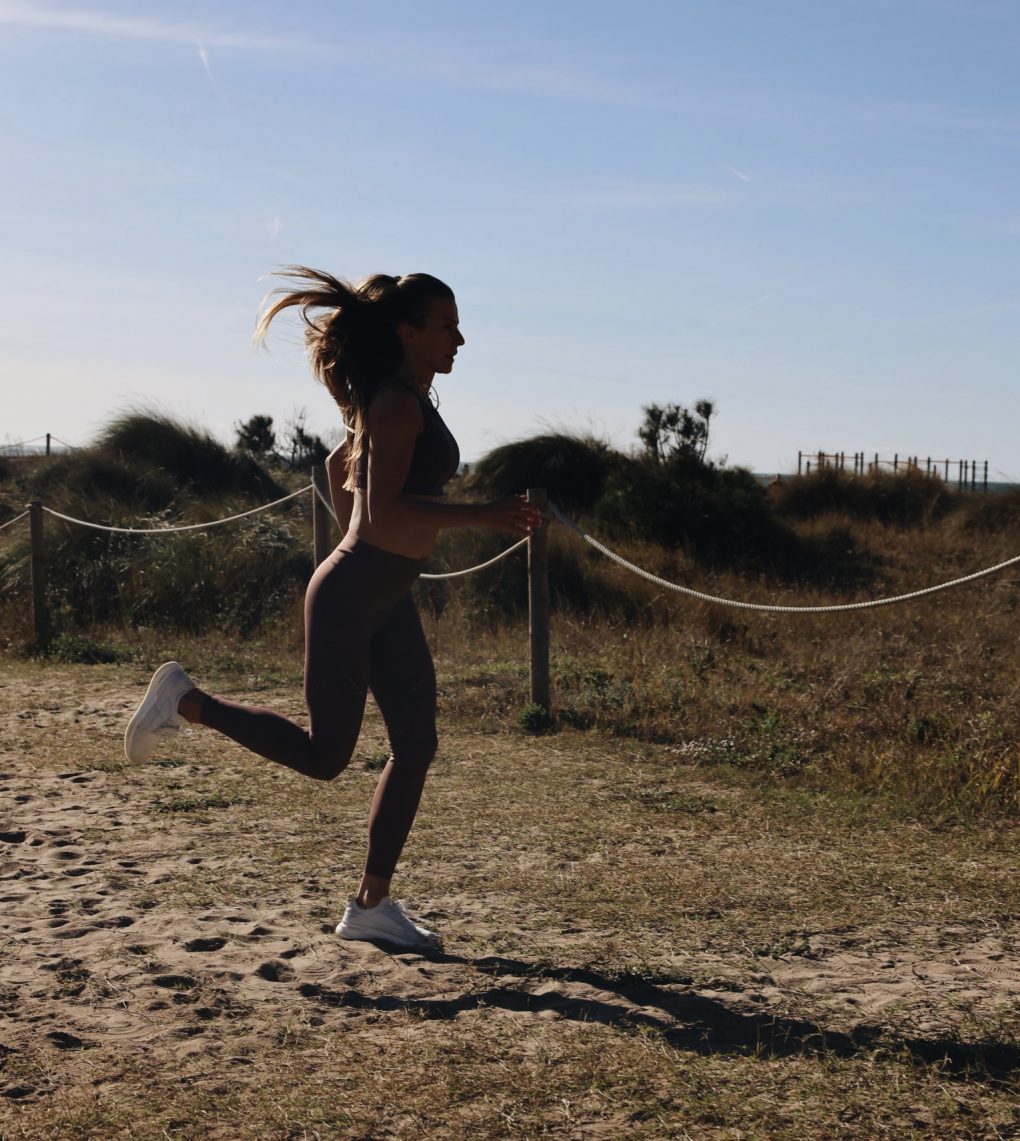In this image, a woman is captured mid-run along a sandy path that exudes an arid, beach-like atmosphere. She is adorned in a brown sports bra and yoga leggings that rise to her belly button, accompanied by white tennis shoes. Her left foot firmly plants on the ground while her right foot is lifted, creating a dynamic portrayal of her motion. Her long hair, likely tied back into a ponytail, flutters with her movement, though her facial features remain obscured by the low, striking sunlight.

The path she runs on is predominantly sandy, flanked by patches of dead, brown grass. A rustic rope fence, tied to wooden poles, delineates the pathway and adds to the natural, rugged landscape. The backdrop features a small embankment overrun with dense brush and grasses, and the tops of palm trees peek out towards the right side of the frame. The sky overhead is blue, accented with faint streaks of clouds, suggesting a bright, clear day. The area has an arid, beach-like feel, possibly with a glimpse of the ocean in the distance, enhancing the overall serene yet vibrant ambiance of the scene.